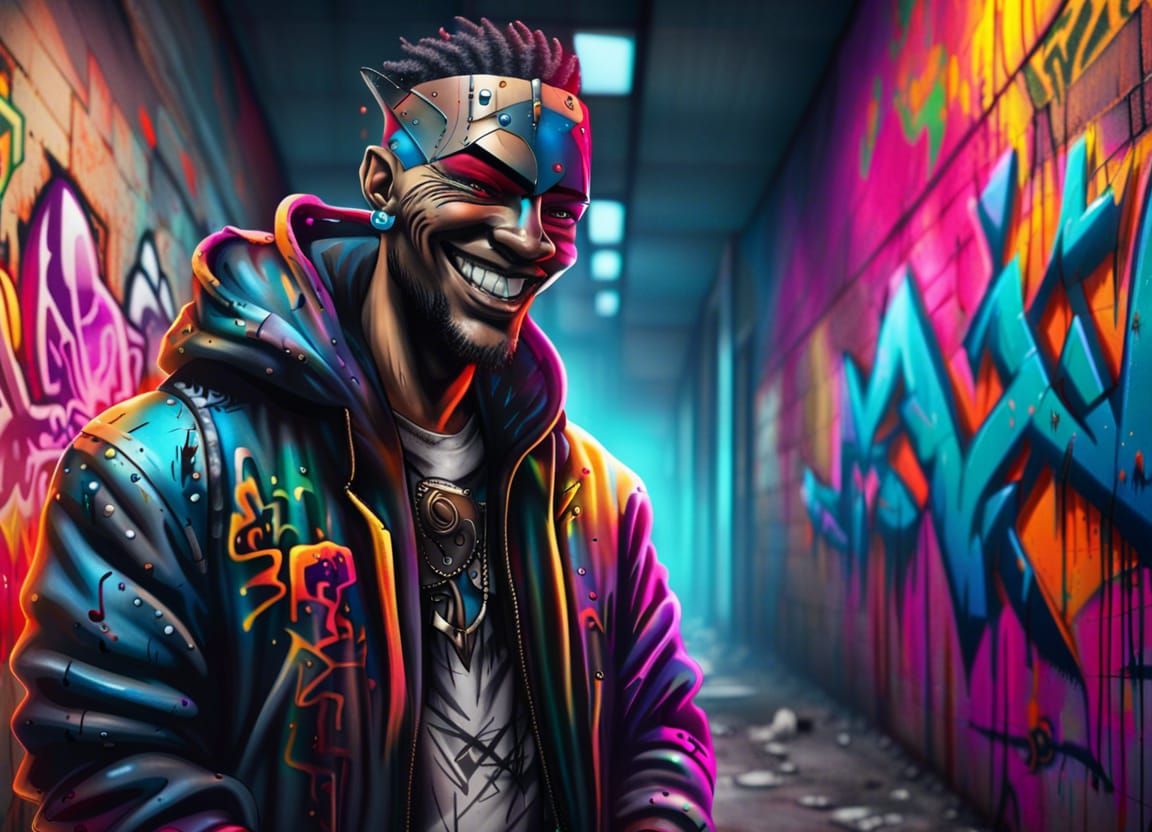In this vibrant, neon-infused digital painting, a black man with spiky black hair and a large, bright smile reveals his striking white teeth, distinctively featuring green lines between them. His forehead is adorned with a metallic headpiece built from interconnected plates in blue, orange, light-colored, and pink hues, fastened with visible tiny screws. He sports a goatee and wears an eye-catching, shiny jacket with textured, wrinkled arms, stained in an array of orange, yellow, pink, and dark blue shapes. Underneath the jacket, a white shirt with an unusual central design peeks out. The scene is set within a vividly colorful environment, possibly a hallway or corner of a building littered with garbage, characterized by light brick walls decorated with unidentifiable neon graffiti in shades of pink, blue, orange, and green. Neon signage adds to the dynamic backdrop, casting an otherworldly glow alongside ceiling lights that illuminate the path ahead. The light blue foggy background further enhances the electrifying and chaotic ambiance.